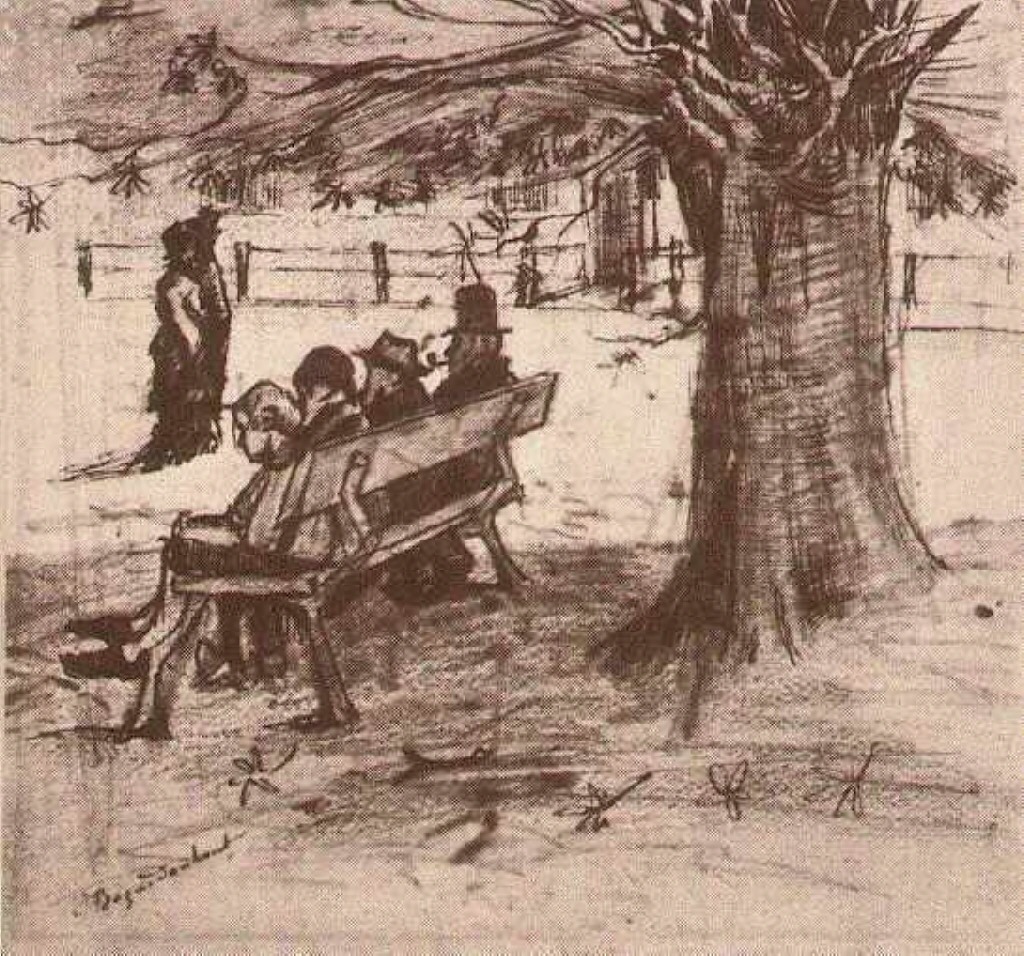The image depicts a detailed hand-drawn charcoal pencil artwork set in a winter-themed park area. At the forefront is a wooden bench with four people, two men and two women from the 18th century, with one man smoking a chrome-covered pipe. Behind the bench stands a towering tree with sprawling branches and sporadic leaves. To the right of the bench, a couple, including a man in a top hat and a woman, can be seen standing. In the background, a long wooden fence and additional trees stretch across the scene, adding depth. The drawing, known for its intricate shading and sketch-like style, also features subtle details such as possible flowers and grass on the ground, and a bird perched on the fence. The artist’s signature is located in the bottom left corner.